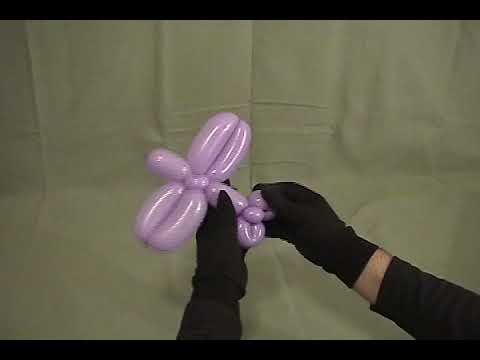In this photograph, a person is skillfully creating a balloon toy that resembles an airplane. The central focus of the image is a long, violet balloon being expertly twisted and folded. The balloon, which exudes a glossy sheen as if illuminated by a light source, is positioned prominently in the center. The hands holding the balloon are clad in black gloves, and traces of a black long-sleeve t-shirt are visible, though only the hands and part of the sleeves are partially seen. A glimpse of a light-complected, hairy arm can be spotted between the glove and the sleeve. The backdrop of the image features a light gray, cloth-like material, possibly a tablecloth, with noticeable wrinkles. Adding to the composition, thin black horizontal strips frame the top and bottom of the image, whereas the sides remain unobstructed. The photograph captures the intricate details and the moment of crafting the vibrant balloon toy against the subdued background.